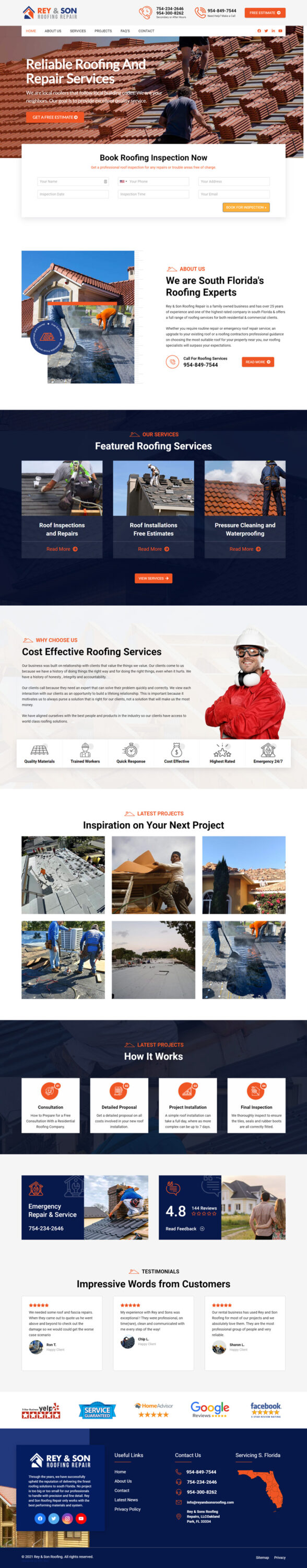The image is a vertically elongated screenshot of a webpage, causing most of the text to appear distorted and unreadable. At the top of the page, the heading "Reliable Roofing and Repair Services" is clearly visible. The webpage features several roof images and is divided into distinct sections. 

The first section emphasizes that the company is "South Florida's Roofing Experts." Following that, there is a section highlighting "Featured Roofing Services." Beneath this section, a light gray background introduces "Cost-Effective Roofing Services."

Further down, the page showcases a gallery of images arranged in two rows with three images each, under the header "Inspiration for Your Next Project." Below this display, there is a blue horizontal background with the title "How It Works," accompanied by four side-by-side boxes with white backgrounds, detailing different aspects of the company's process.

An area with customer feedback is indicated by a visible rating of 4.8 stars, although its authenticity is uncertain. Finally, there is a section labeled "Impressive Words from Customers," featuring three horizontally aligned, white rectangular boxes, presumably containing customer reviews.